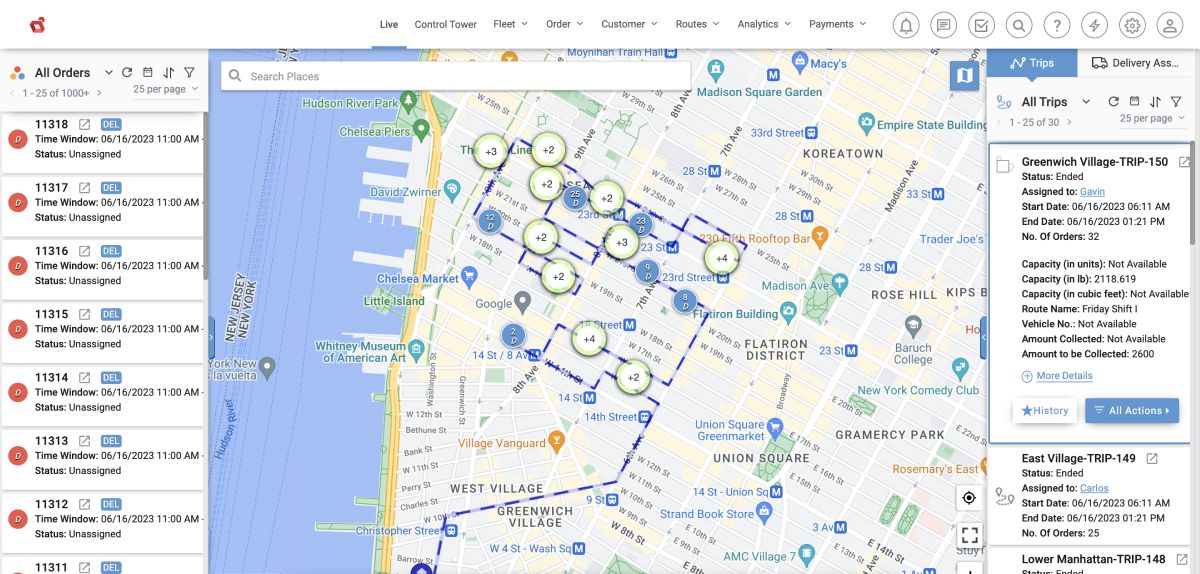This image is a screenshot of a logistics management software interface, which is approximately two and a half times wider than it is tall. The top center features a navigation menu with options such as "Live," "Control Tower," "Fleet," "Order," "Customer," "Routes," "Analytics," and "Payments," all presented in black text on a white background. To the right of this menu, there are several clickable icons, including a bell, chat window, box with a check mark, magnifying glass, question mark, lightning bolt, gear, and a person icon.

On the left-hand side of the interface, there is a vertical column labeled "All Orders." This column lists five-digit order numbers (e.g., 11318), along with corresponding details such as "Time Window," "Status," and "On a Sign." Seven orders are fully visible, and an eighth is partially cut off at the bottom of the column.

Occupying about two-thirds of the central area is a detailed map marked with various pins, indicating different locations or deliveries. On the right-hand side of the interface, there is a section resembling an email inbox, displaying headers, dates, times, and titles, likely providing more detailed information for each order.